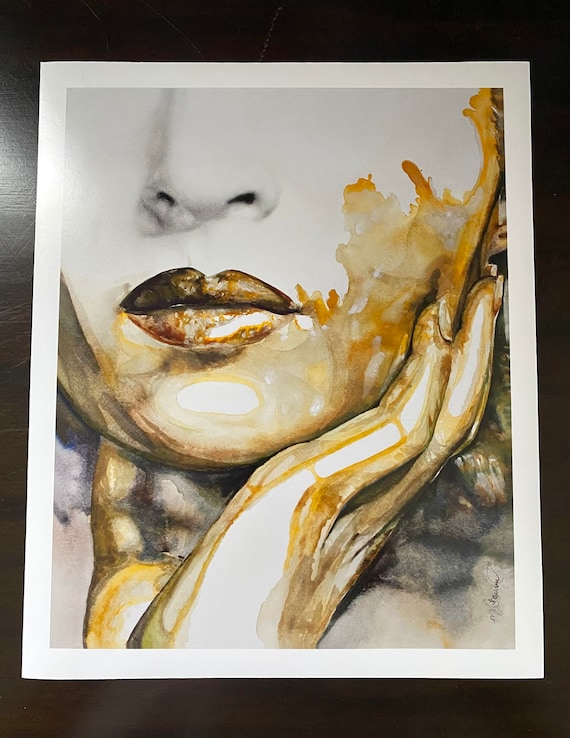This piece of artwork is a captivating illustration of a female-presenting model, focusing exclusively on the area from her nose down. The image combines elements of drawing and painting, blending pencil-like detail on the nose with watercolor or possibly coffee-based hues on the lips, chin, cheeks, and hands. The model’s porcelain-like skin contrasts with the golden and orangey-brown pigments that splash across her lips and cheeks, creating an intriguing juxtaposition. Her hand, adorned with visible fingernails, gently cups her chin, adding a sense of contemplative calm. The golden and burnt orange smears extend over her face and hand, enhancing the texture and depth of the image. The lower part of the painting is more blurred, with a smeared effect that further enriches the visual complexity. All of this is set against a minimalist, gray and black background and framed within a white border, resting on a black surface.